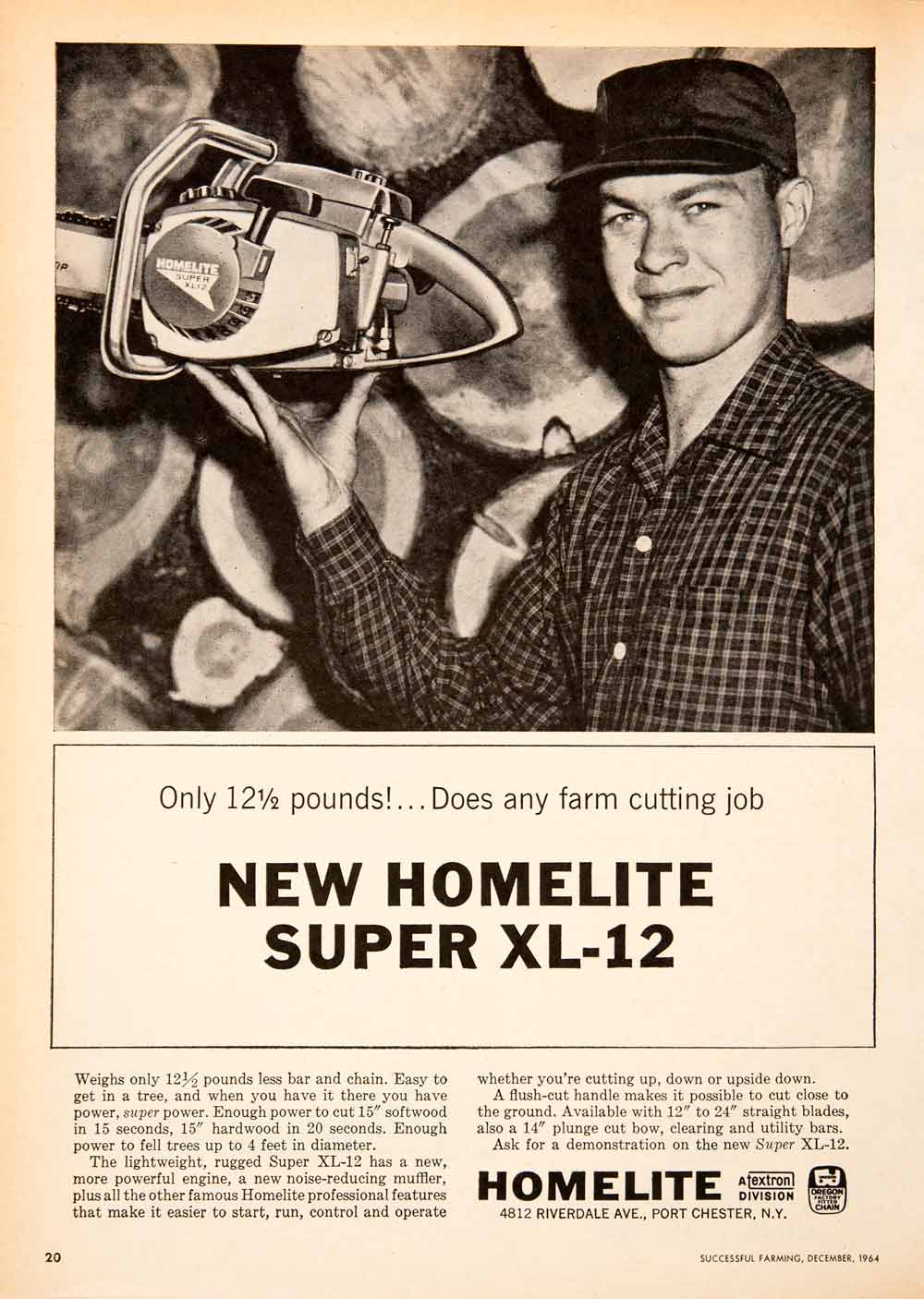This vintage black and white poster, printed on aged, tan-colored paper, is divided into three sections. The upper section features a Caucasian man wearing a plaid shirt and a cap with the bill facing forward. With a small, closed-mouth smile, he holds the end of a silver chainsaw, identifiable as motorized, delicately with his fingertips. Behind him, stacks of firewood are visible. Below his image, a prominent black box contains text in various fonts: "Only twelve and a half pounds! ... does any farm cutting job." In bold, large letters, it reads "NEW HOMELITE Super XL-12." The bottom section of the poster includes multiple paragraphs of small print text, with the word "Homelite" noticeably larger in black font, accompanied by an address: 4812 Riverdale Ave, Port Chester, New York. The aged page's slight yellowish-white tint complements the overall vintage aesthetic.